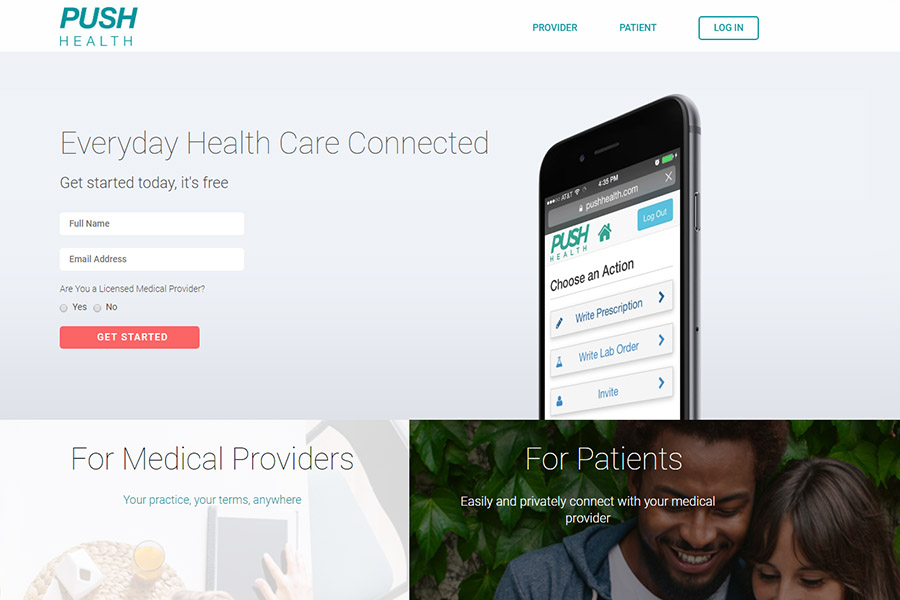The image depicts a website layout with distinct design elements and informational sections. 

At the very top of the page, occupying approximately the first 10% of the vertical space, the background is white. On the upper left corner, there is teal-colored text that forms the site's logo. The text "Push" is bold, larger in font, and italicized, while "Health" is written below it in a regular font style. Moving to the upper right-hand side, there are three menu options: "Provider," "Patient," and "Login." The "Login" option is highlighted with a rectangular button surrounding it.

Below this white header, the background shifts to a light gray for roughly the next 60% of the vertical space. On the left-hand side, there is a prominent heading in large font with the first letter of each word capitalized: "Every Day Healthcare Connected." Below this headline is a smaller-font message in the same color, stating, "Get Started Today. It's free." Beneath this message are two input fields with a white background, labeled "Full Name" and "Email Address." Additionally, there are checkboxes for "Are You a Licensed Medical Provider?" with options for "Yes" or "No." A red "Get Started" button completes this section.

On the right side of this gray-background area, an image of a smartphone displays the app interface of the website. Further down, the page is divided into two sections titled "For Medical Providers" and "For Patients," likely offering more detailed information or links tailored to each group.